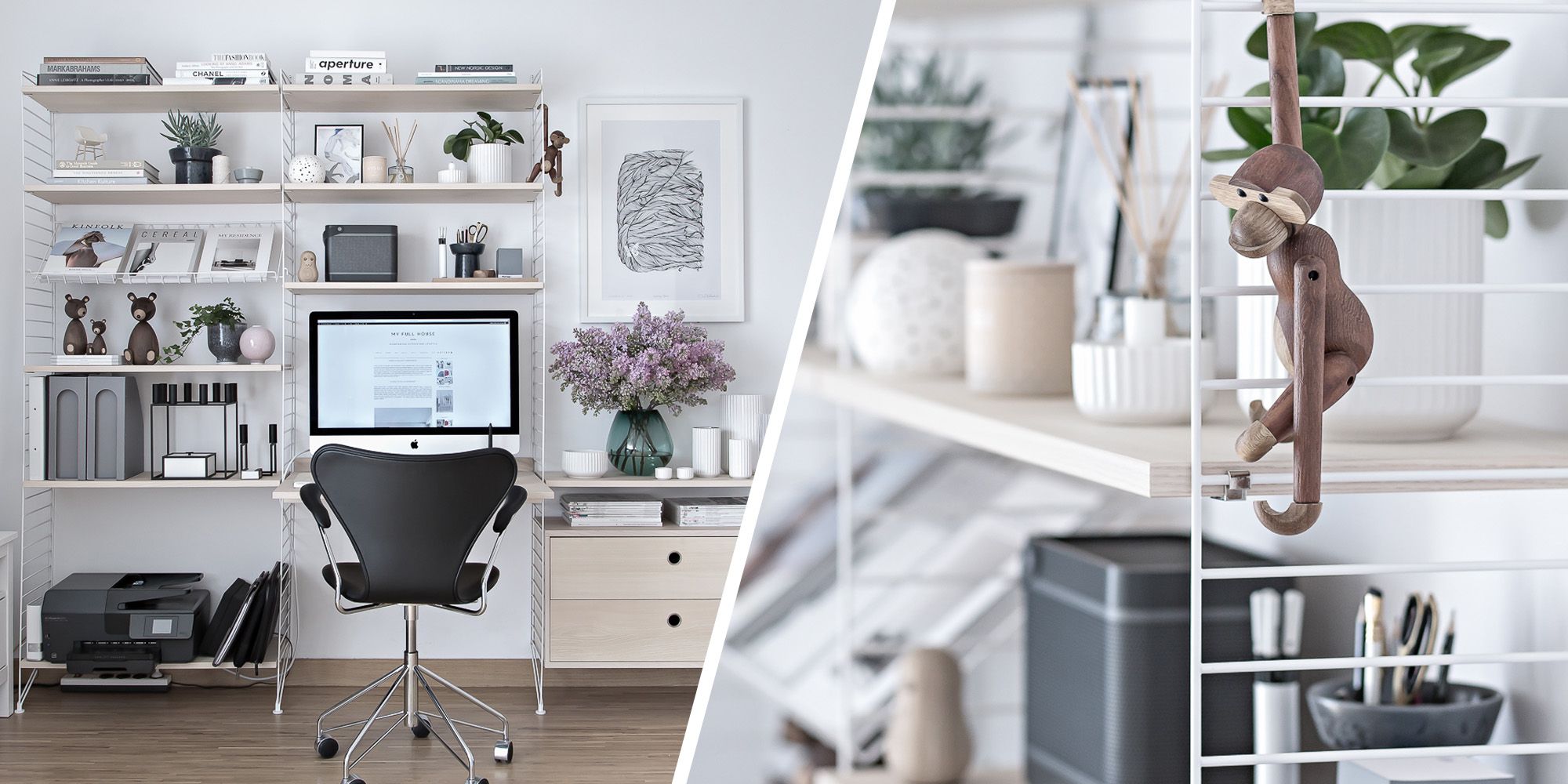The image is split diagonally into two sections, both depicting a meticulously organized and stylish office space. The left side of the photo offers a full view of a white room dominated by a metal and light wood combination desk that also functions as a bookshelf. The desk is just large enough to support a monitor and an adjacent black office chair with silver legs and wheel casters. The bookshelf displays a blend of functional items and decorative pieces: on the lowest shelf sits a printer, while the upper shelves house file folder holders, various books, framed photographs, decorative little bear statues, and potted plants. Notably, there is a small wooden monkey hanging from the wire side of the bookcase, a detail that's more closely captured in the right side of the photo. The top shelf also includes more books and stationery items such as a cup of pens.

To the right of the desk, there is a small end stand with two drawers. Atop this stand, there is a green vase containing purple flowers, some white candles, and a white bowl. Positioned against the white wall, this end stand also features an abstract black and white sketch in a frame. The close-up on the right zooms in on the side of the bookshelf, highlighting the wire structure that allows visibility through to the white and cream-colored objects within, including more green plants. Prominently hanging on the side of the wire bookshelf is a wooden monkey and a small piece of decorative art, echoing the office's thematic use of natural and artistic elements.